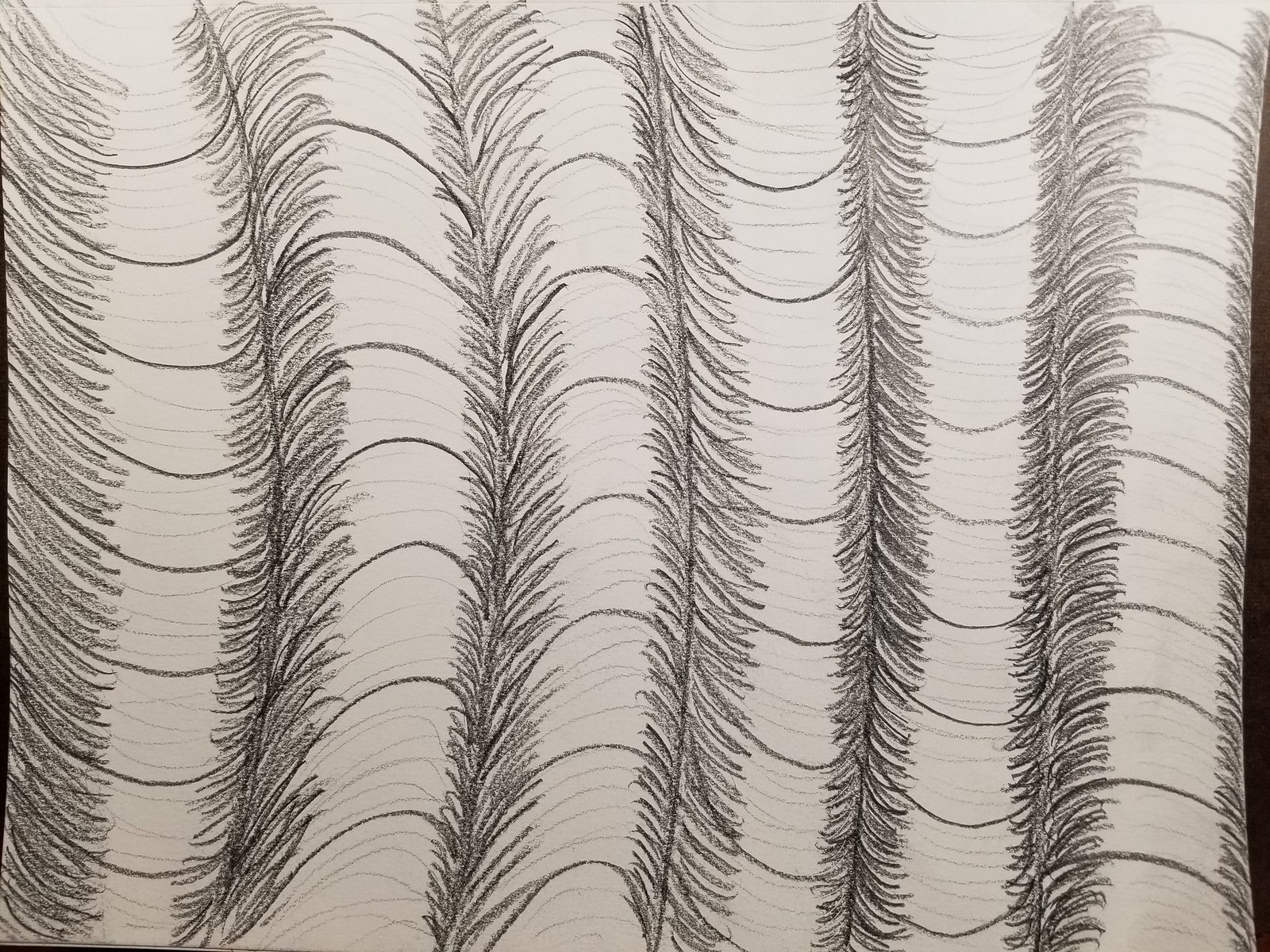Here we have an intricately detailed pencil drawing featuring six vertical, cylindrical forms, each resembling metal tubes sectioned off by horizontal lines at regular intervals, suggesting potential points of flexibility. The tubes are primarily white at the top, transitioning into a shaded gray-black on the sides, achieved through repetitive pencil strokes. This meticulous shading technique creates a textured, three-dimensional effect, enhancing the perceived depth and curvature of the tubes. The parallel, scratch-like marks on the sides further emphasize the rounded edges of the design, lending a sense of realism and volume to the image.